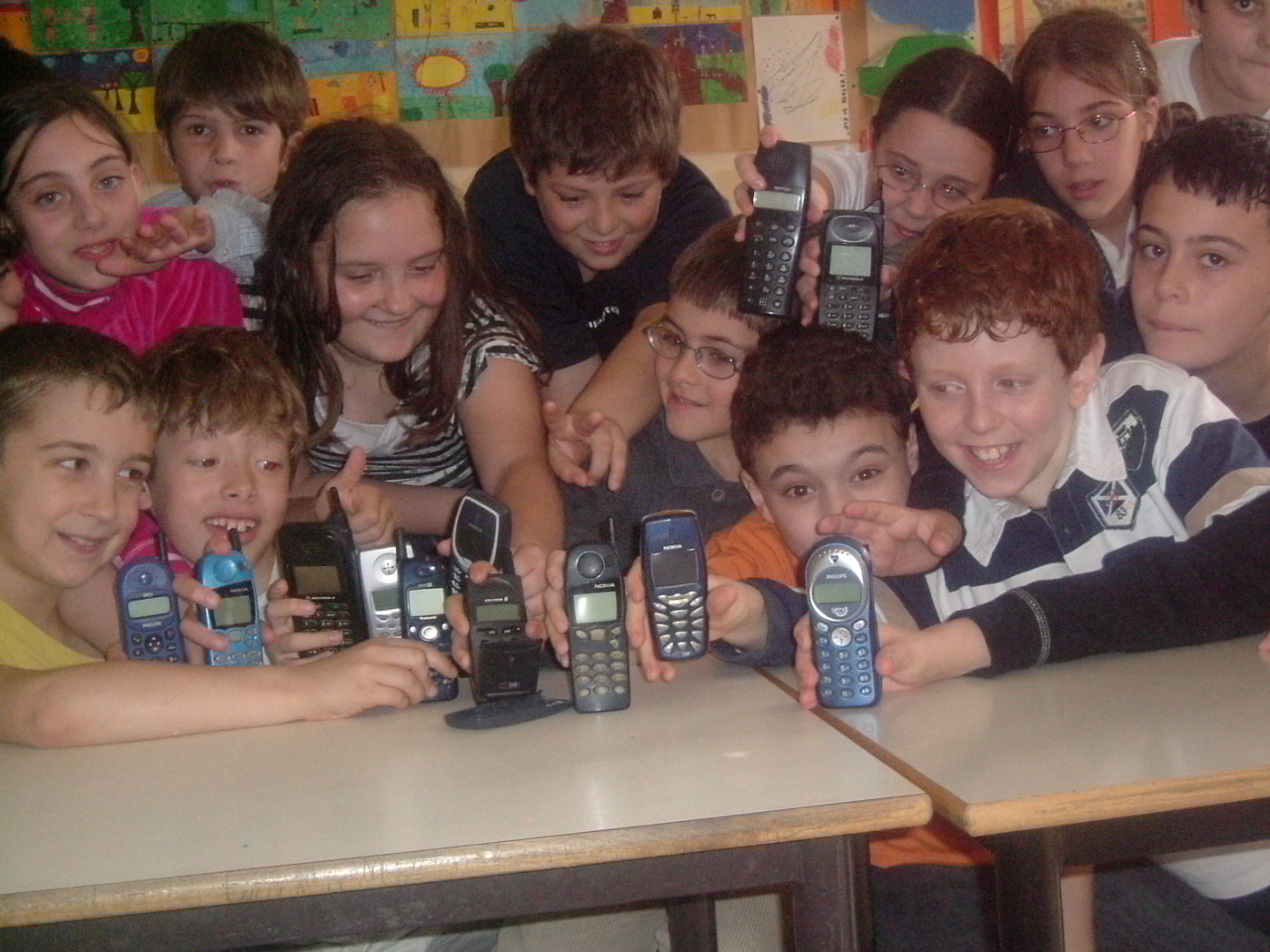A color photograph captures a lively group of twelve elementary school children, likely fourth grade and above, gathered in a classroom behind two light brown wooden desks. They are all Caucasian, smiling joyfully and holding eleven old-school cell phones, reminiscent of earlier models like Nokia, with small digital screens and physical buttons instead of the modern touchscreen. The children are a mix of boys and girls, appearing from the chest up as they pose with their antique devices. In the background, the classroom is adorned with a bulletin board showcasing vibrant, child-made artwork depicting a blue sky and trees, adding a creative and cheerful atmosphere to the scene.